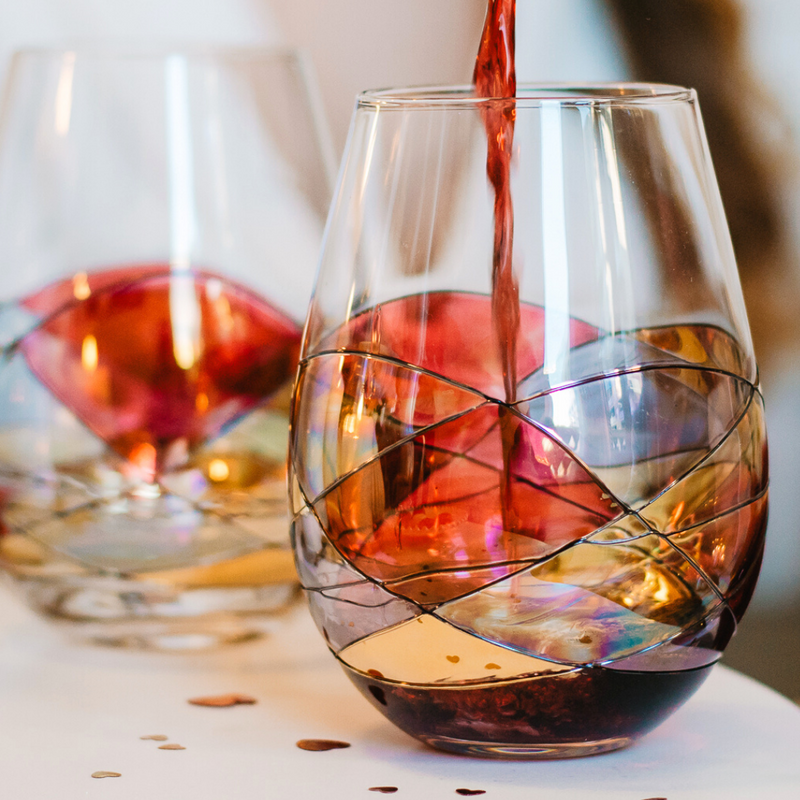In this vivid close-up color photograph, red wine is being elegantly poured into a unique stemless glass adorned with a stained glass-like design in harmonious shades of red, yellow, and blue. The glass, though colorful, retains a translucent quality, allowing the light to gently pass through and create a soft, almost ethereal glow. As the wine enters the glass, it begins to fill the bottom, highlighting the intricate patterns. Positioned on a pristine white tablecloth, the scene includes small drops of red wine scattered across the surface, adding a casual touch to the setting. Behind the primary glass, another similarly designed but empty stemless glass stands slightly out of focus, receiving a subtle glare from the ambient light. The background remains blurred, ensuring the colorful focal point remains sharply defined and eye-catching.